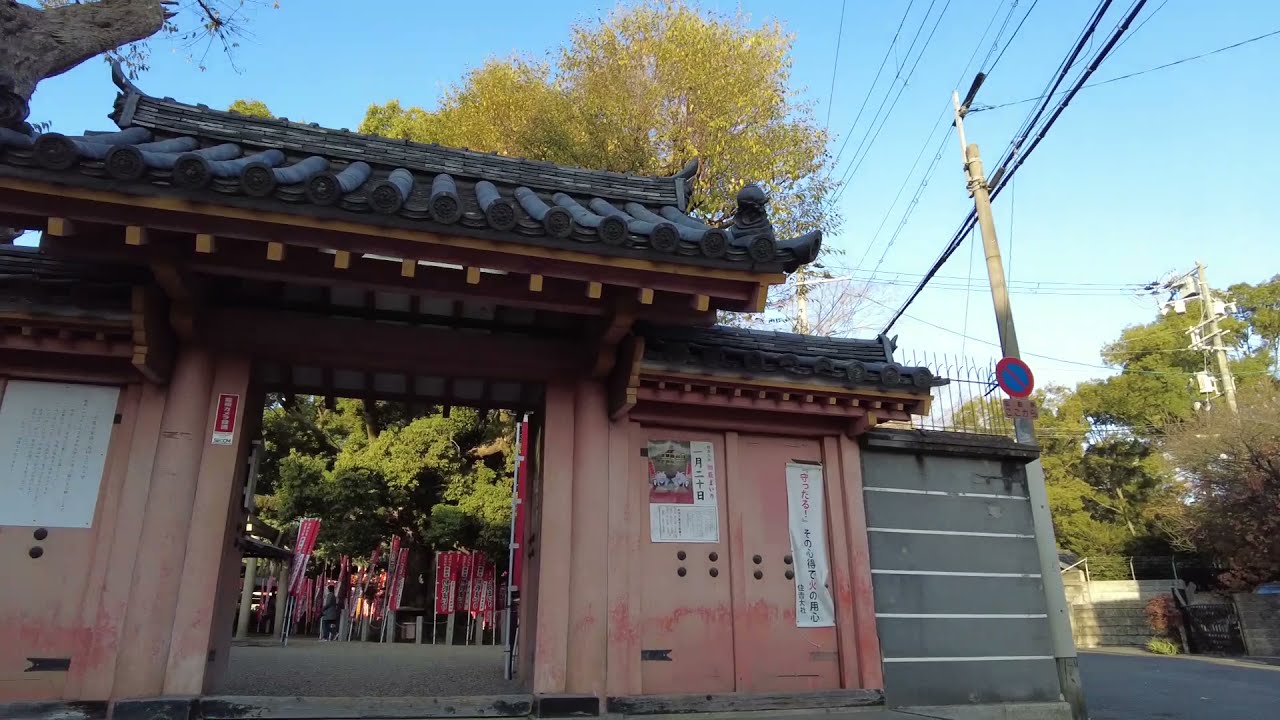The image captures the entrance of an old-fashioned Japanese house made of light brown and light red wood, adorned with a traditional dark, layered tile roof with upturned corners. Through the doorway, you catch a glimpse of a courtyard filled with vibrant red banners. On the right side of the entrance, two posters with Japanese characters are affixed to the wall, while a white plaque with additional writing is seen on the left. The building’s once-vibrant pink or red paint has faded, although brighter patches remain. Above the roof, a large tree extends its branches, framing a clear, bright blue sky interrupted by numerous overhead power lines. To the right, a section of the road is visible along with additional trees and a "Do Not Enter" sign hanging from a light post.